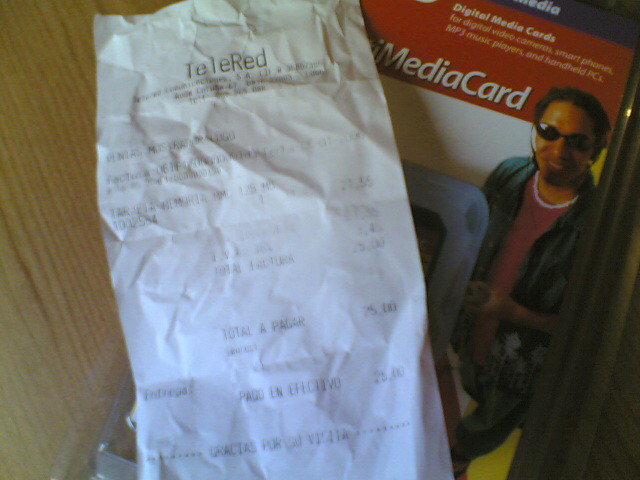On a tabletop, there are two items captured in this image. The first item is a plastic container designed to hold media cards, specifically for digital devices like video cameras, smartphones, MP3 music players, and handheld PCs. The case is predominantly white, with a red top portion. Adorning the case is an image of a man sporting sunglasses, an unbuttoned shirt, and a white or possibly coral necklace, adding a vibrant and casual look to the packaging. The second item is a crumpled receipt, likely confirming the purchase of the media card. Though the receipt is difficult to read due to its condition, the visible text indicates it is written in Spanish, featuring the phrase "gracias por," which translates to "thank you for" in English.